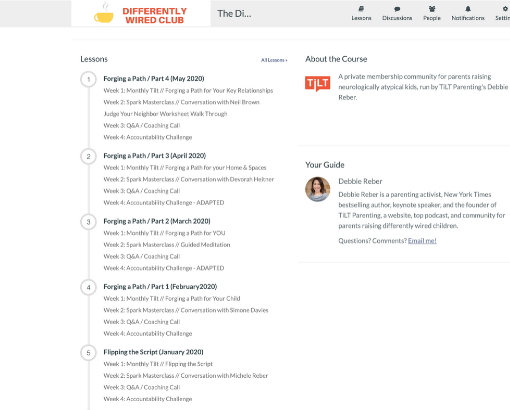This image is a screenshot of a website with a predominantly white background. At the top, there is a gray navigation bar featuring an orange logo that reads "Wired Club." To the left of the logo, there is an icon of a yellow coffee cup. Over to the right side of the bar, there are five icons, each paired with text below them.

Below the navigation bar, the main content of the page is divided into two sections. On the left side, there's a list of five lessons. Each lesson entry includes a title, the dates of the course, and subtitles for weeks one through four. Four of the lessons are part of a series titled "Forging a Path," with the descriptions listed as part one through four. The final lesson is titled "Flipping the Script."

On the right side of the page, there is a section labeled "About the Course," which provides an overview of the course content. Directly below this, there is a section named "Your Guide," which presumably offers information about the course instructor or mentor.